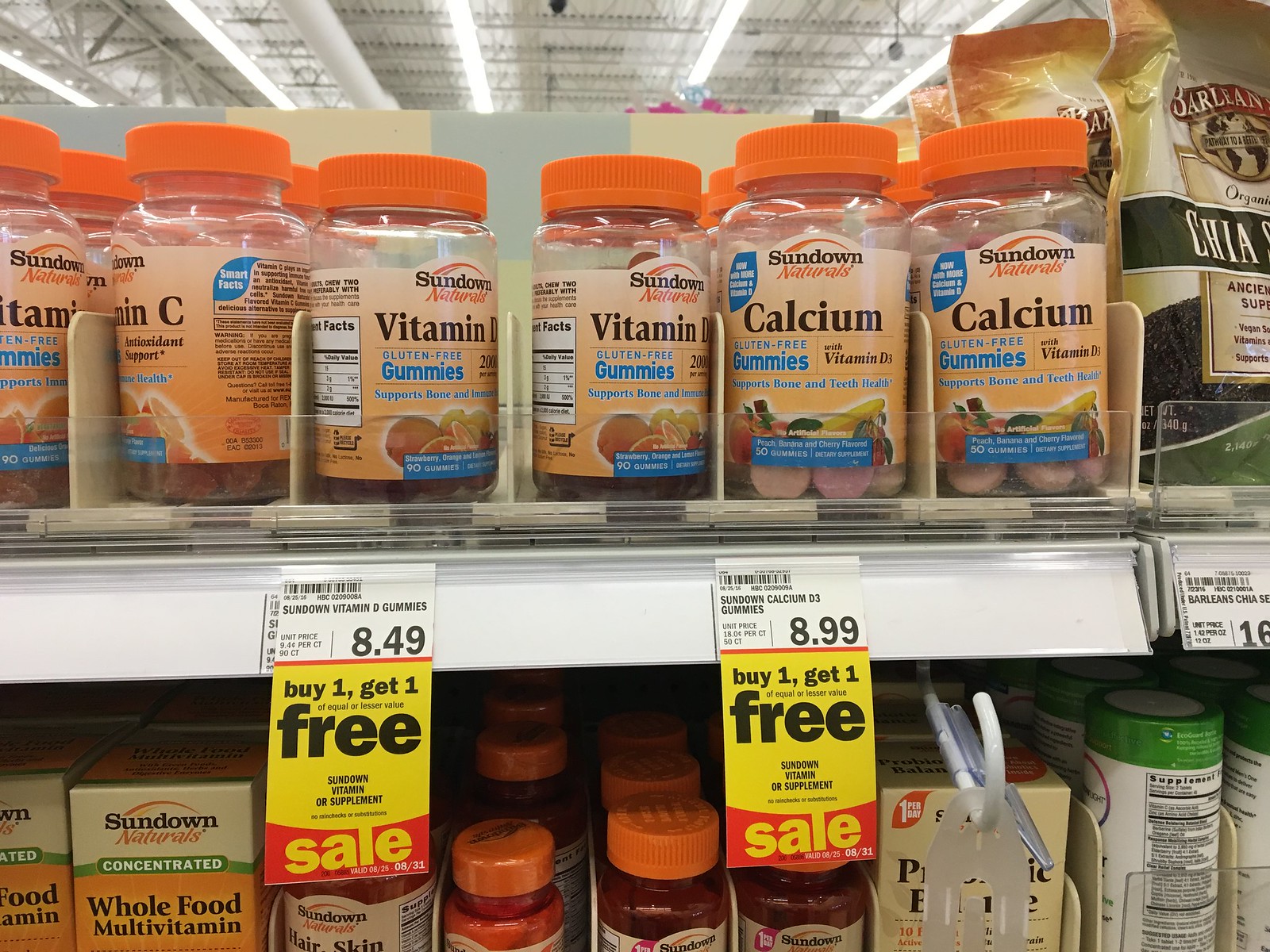The image captures an interior view of a store with two prominent white shelves. On the top shelf, there's a variety of Sundown Naturals vitamin products. To the left, there are two jars of Vitamin C with clear containers and orange tops. Adjacent to these, two rows of Vitamin D gummies in clear containers with red lids are displayed, with a price tag of $8.49 and a "buy one, get one free" sign. Next to the Vitamin D gummies are bottles of calcium gummies, also by Sundown Naturals, similarly packaged in clear bottles with orange tops. A bag of chia seeds rests nearby. The bottom shelf mainly shows the tops of various vitamin jars, some with bright orange caps, including a Sundown Naturals whole food multivitamin box with a white top, green line, and orange bottom. Additional jars with green lids and a tan box are seen to the right. The background features a pattern of tan, yellow, and gray squares, with a glimpse of the ceiling at the top of the image.